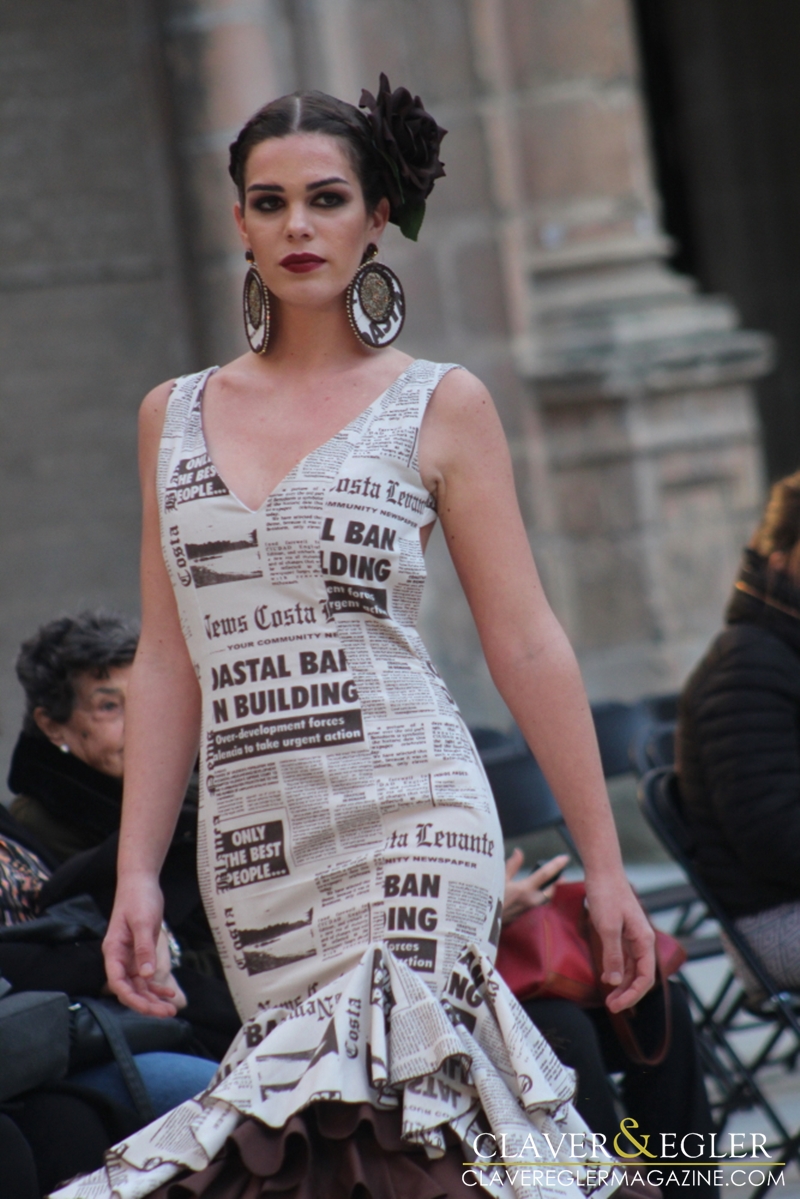This photograph captures a striking scene, likely from a modeling show, set in an outdoor location. The focal point is a woman embodying avant-garde fashion. She is styled with her hair up, adorned with a prominent black flower on the side of her head, and wears large hoop earrings that graze her shoulders. Her dress, a tight, sleeveless creation with a v-neck that hugs her form down to her thighs before flaring out in a ruffle, is uniquely designed with a black and white newspaper print, featuring various headings and articles. In the background, a brick wall and several seated people, some dressed in mink or fur coats, are visible, adding to the scene's layered ambiance. At the bottom right corner of the image, text reads, "clever and regular, a CLA, a Virgil or magazine dot com," further hinting at the fashionable context of the photograph.